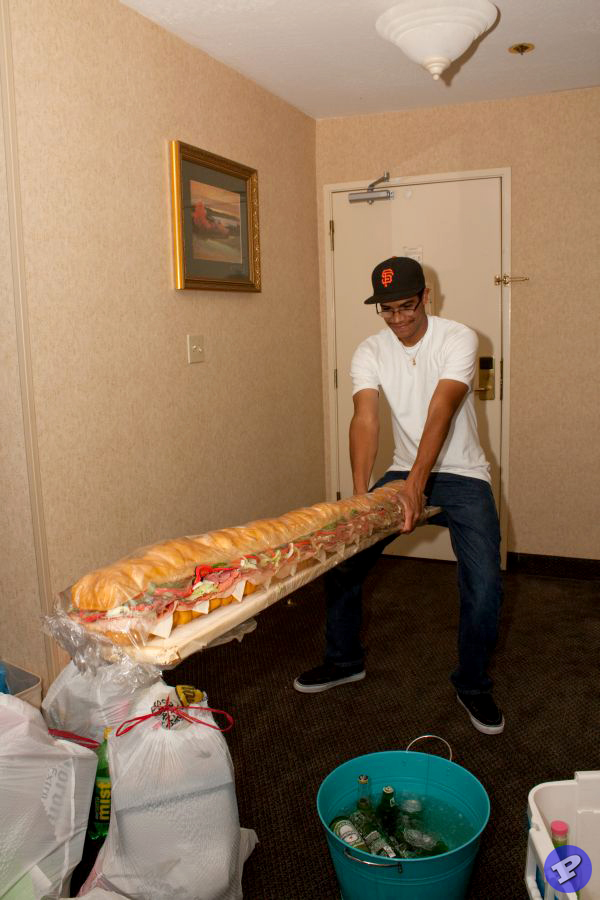This detailed image shows a man standing in what appears to be a hotel room. The room features a white door with an extra security lock and deadbolt, a framed photo with a gold frame and green border, and a reddish-pink wall. The floor is covered with a brown carpet, and there are several trash bags scattered around.

The man has dark brown skin and is dressed in a white t-shirt, blue jeans, black sneakers with white soles, and a gold necklace. He also wears glasses and a black San Francisco Giants baseball cap with a red symbol in the middle. He is holding an enormous hoagie sandwich, approximately six to ten feet long, filled with various types of meats, cheeses, lettuce, tomatoes, and other vegetables.

On the floor beside him, there’s a blue bucket filled with ice and bottles of beer, and next to it is a cooler containing a bottle with a pink cap. Additionally, there's a purple stamp with the letter "P" in it, visible on the carpet.